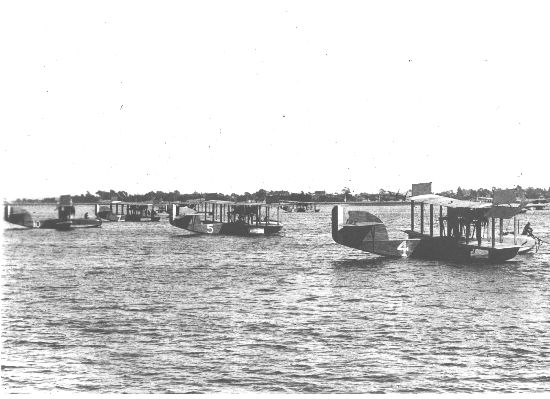This black-and-white antique photograph depicts a serene scene of several vintage seaplanes resting motionlessly on a vast body of water. In the foreground, four distinct seaplanes can be seen in alignment, each marked with spray-painted white numbers for identification. The seaplane on the far right bears the number "4," followed leftwards by planes numbered "5," "7," and "10." These seaplanes appear to be constructed from a rudimentary, almost plank-like material, adding to their vintage charm and historical aura. The image, evocative of an earlier era, silently captures these aircraft as they remain afloat. Behind the line of seaplanes, the far background silhouettes what might be distant buildings or a tall tree line, though the details are blurred and ambiguous, adding a sense of mystery due to the photograph’s aged and monochromatic quality.